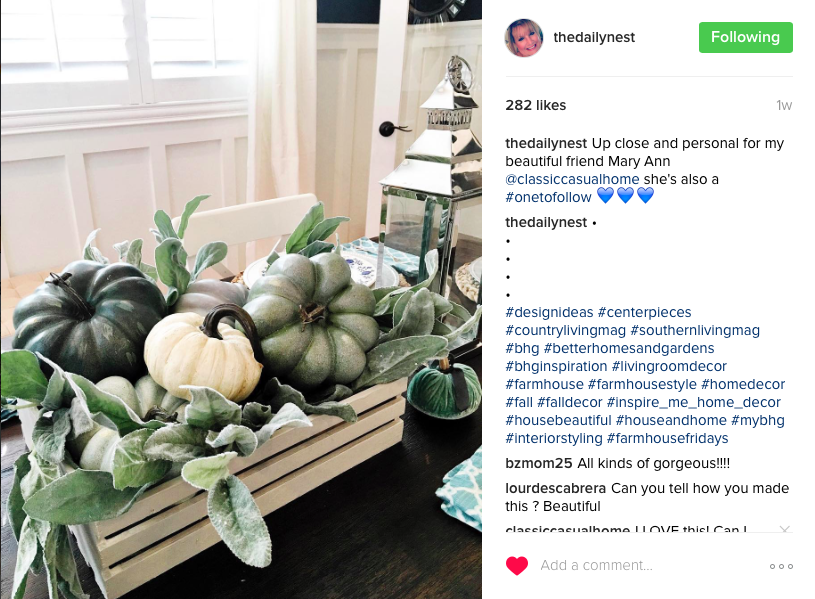The image is a detailed screenshot of an Instagram post by the account "The Daily Nest." The centerpiece of the image is a beautifully arranged tablescape. At the center of the table, there is a white wooden box overflowing with an assortment of small, artificial pumpkins in various colors such as black, gray, light green, and white. Surrounding the box are lush eucalyptus leaves, adding a touch of greenery. To the right of this arrangement stands a large silver lantern, adding an elegant flair to the setting.

The right-hand side of the screenshot features Instagram's interface with a white background. At the top, the account name "The Daily Nest" is prominently displayed. Next to it, a large green bar with the word "Following" indicates that the viewer is following this account. Below this, the post has garnered 282 likes. The caption reads: "Up close and personal for my beautiful friend Mary Ann," followed by a tagged user and the hashtag #onetofollow, suggesting that Mary Ann is a notable person worth following.

Further down, the account name "The Daily Nest" appears again, accompanied by four bullet points, presumably detailing aspects of the post or the account. Beneath these points lie approximately 30 hashtags, strategically used to maximize the post's reach. The section is capped off with various user comments, adding to the engagement and interaction with the post.